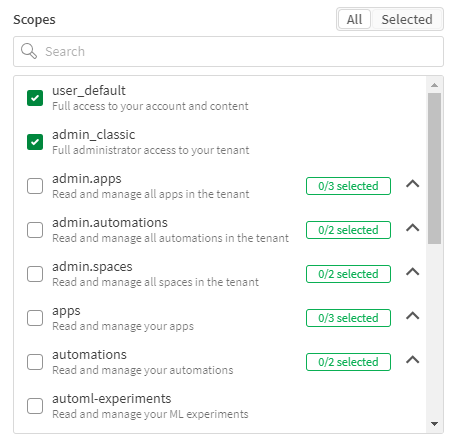This is a cropped screenshot of an admin settings panel from an administrative interface. In the top left corner, the word "Scopes" appears in small black letters. Immediately to the right of "Scopes," there is a thin gray box divided into two sections labeled "All" on the left and "Selected" on the right. The "Selected" option is currently chosen and grayed out, while the "All" option is displayed within a white box.

Directly below this, there is a large search bar stretching across the panel from left to right. Beneath the search bar, there is a wide, square scroll box that includes a visible scroll bar on its far right side, which is currently positioned at the top.

The main content of the scroll box consists of vertical checkboxes aligned along the left side. Each checkbox is associated with a title and a short description displayed to its right. The first entry reads "User Default," and its description states "Full access to your account and content." This checkbox is marked as checked. The second entry is labeled "Admin Classic," with a description that reads "Full administrator access to your tenant." This checkbox is also checked.